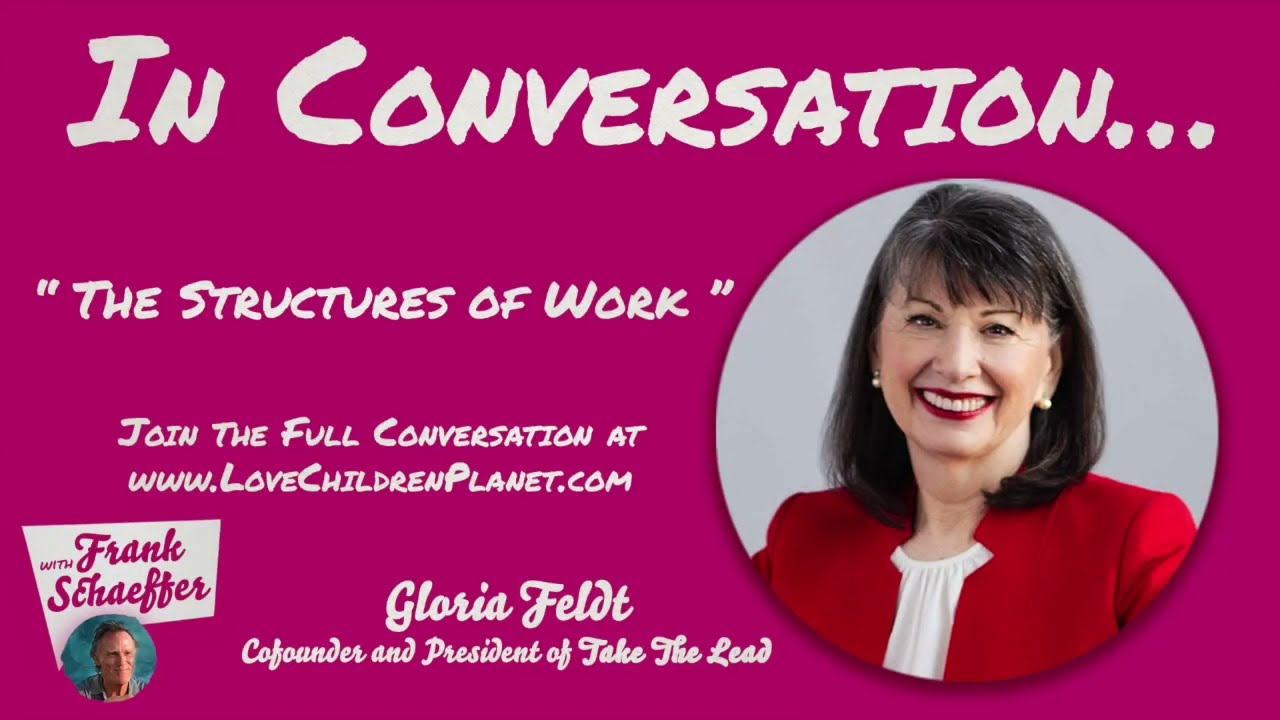The image is a hot pink advertisement for a discussion titled "In Conversation... The Structures of Work," directing viewers to join the full conversation at www.lovechildrenplanet.com. The prominent feature on the right side of the image is a large circular headshot of Gloria Felt, the co-founder and president of Take the Lead. Gloria is smiling, wearing a red suit jacket over a white blouse, with pearl earrings, red lipstick, and gray-streaked dark hair. She has a peach complexion. In the bottom left corner is a much smaller circular headshot of Frank Schaefer, with text above his image indicating his participation in the conversation. Frank has a peach complexion, a gray shirt, and a blue background. The text throughout the image is white, set against the vibrant magenta background, making for a simple, business card-style design aimed at promoting the event.